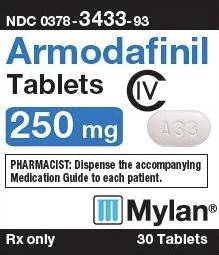The image features a medication known as Armadafinil tablets, prominently displayed with detailed information. The tablets are oval-shaped, white, and have "A33" stamped on one side. They are sold in 250 milligram quantities. The packaging includes a grey panel at the top containing the code "NDC 0378-3433-93," which likely identifies this specific medication. 

Additionally, there's a small grey panel labeled "Rx only, 30 tablets." Below this, another grey rectangle contains a warning for pharmacists, instructing them to dispense the accompanying medication guide to each patient.

The name brand "Armadafinil" is written in blue against a white background, directly beside the tablet. Beneath the brand name, the word "tablets" appears in black text. "250 mg" is highlighted in white text within a blue rectangle. 

The manufacturer, Mylan, whose name is a registered trademark, produces this medication.